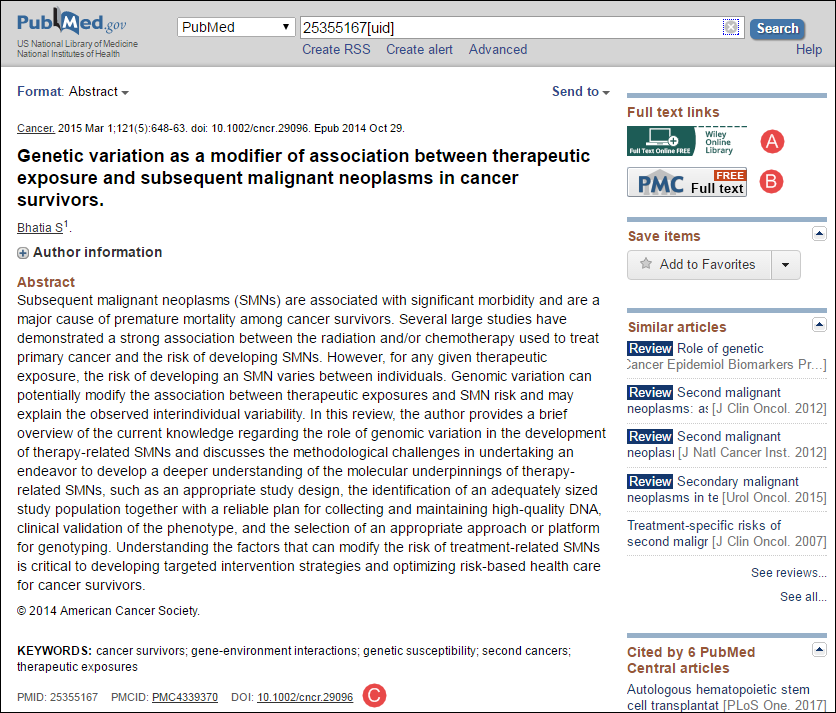Screenshot of a PubMed Page Detailing Search Results for a Genetic Variation Study in Cancer Survivors

This square-shaped screenshot captures a page from PubMed, a database of biomedical literature. At the top, a horizontal gray banner spans the page, with "PubMed.gov" displayed prominently in blue text on the upper left-hand corner. Below this, in finer gray text, it reads "U.S. National Library of Medicine, National Institutes of Health." The header includes a dropdown menu labeled "PubMed" positioned centrally, and a search bar below it displaying the query "25355167 [UID]" enclosed in brackets. To the right, there is an oval blue button with the word "Help" inscribed in gray text. Adjacent to it on the right is another blue button labeled "Search."

Beneath these menu options, the page transitions to a clean white background displaying search results. The first notable result is an article citation from the journal "Cancer," dated March 1, 2015, appearing in volume 121, issue 5, on pages 648-663. The DOI for the article is "10.1002/CNCR.29096," and the article was electronically published on October 29, 2014. The study focuses on the role of genetic variation as a modifier in the association between therapeutic exposure and the development of subsequent malignant neoplasms in cancer survivors.